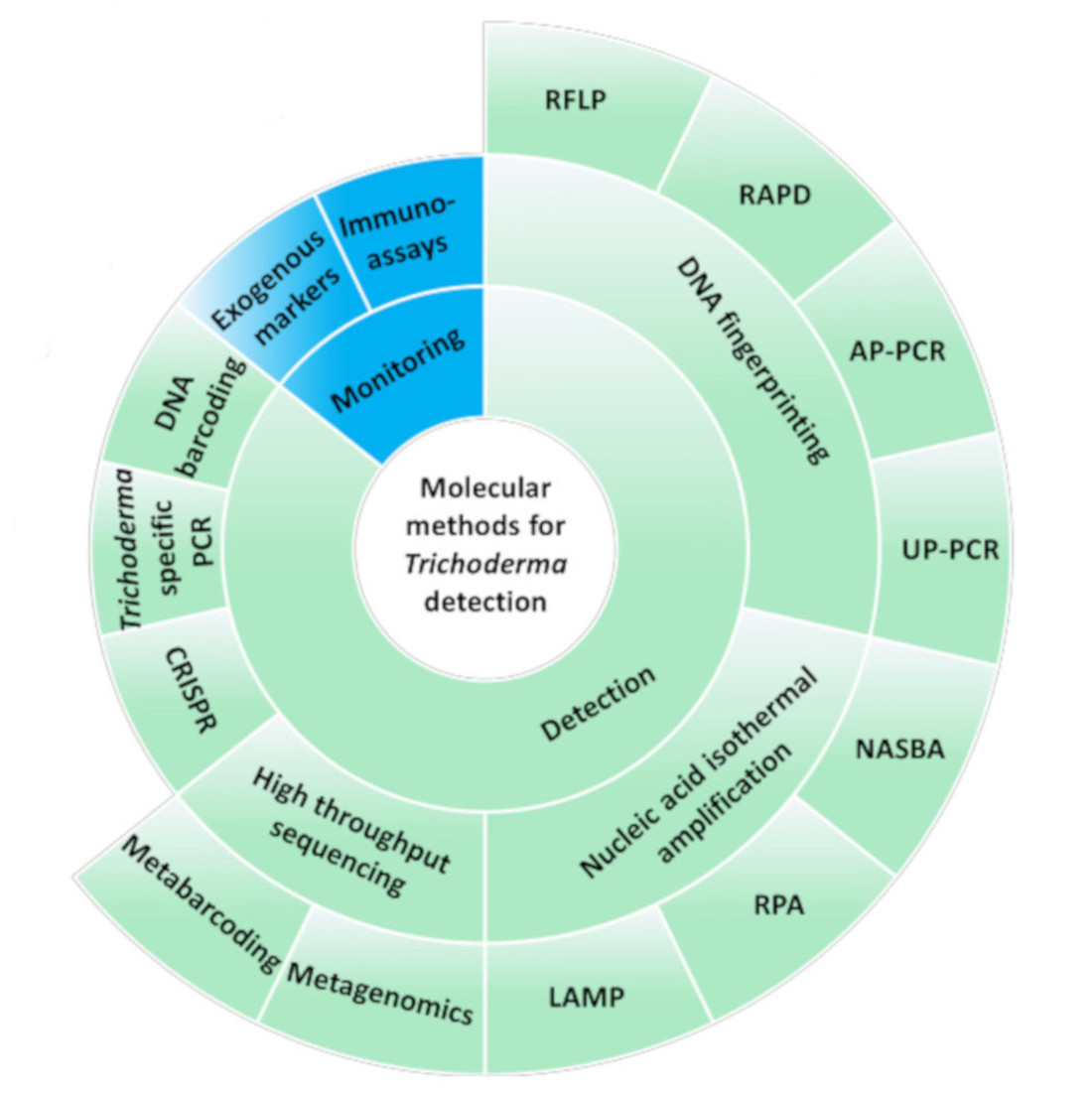This infographic appears to be from a science textbook and is designed to illustrate molecular methods for Trichoderma detection. The diagram is predominantly circular and spiral-shaped, set against a white background. At the center, a white circle contains the text "Molecular Methods for Trichoderma Detection" in black. Surrounding this central circle are concentric circular sections, resembling a pie chart.

The next layer is principally green and labeled "Detection," whereas a smaller adjacent segment is blue and labeled "Monitoring." Extending outwards, additional blue sections labeled "Exogenous Markers" and "Immunoassays" are connected to the monitoring segment. 

Further out in the green detection area, terms such as "DNA Fingerprinting," "Nucleic Acid Isothermal Amplification," "High-Throughput Sequencing," "CRISPR," "Trichoderma-Specific PCR," and "DNA Barcoding" are featured. Subcategories linked to DNA Fingerprinting include "RFLP," "RAPD," "AP-PCR," and "UP-PCR." The isothermal amplification section connects to "NASBA," "RPA," and "LAMP," while the high-throughput sequencing area includes "Metabarcoding" and "Metagenomics."

Overall, the infographic is detailed and text-heavy, visually structured to categorize and differentiate various molecular methods and technologies used for detecting Trichoderma.